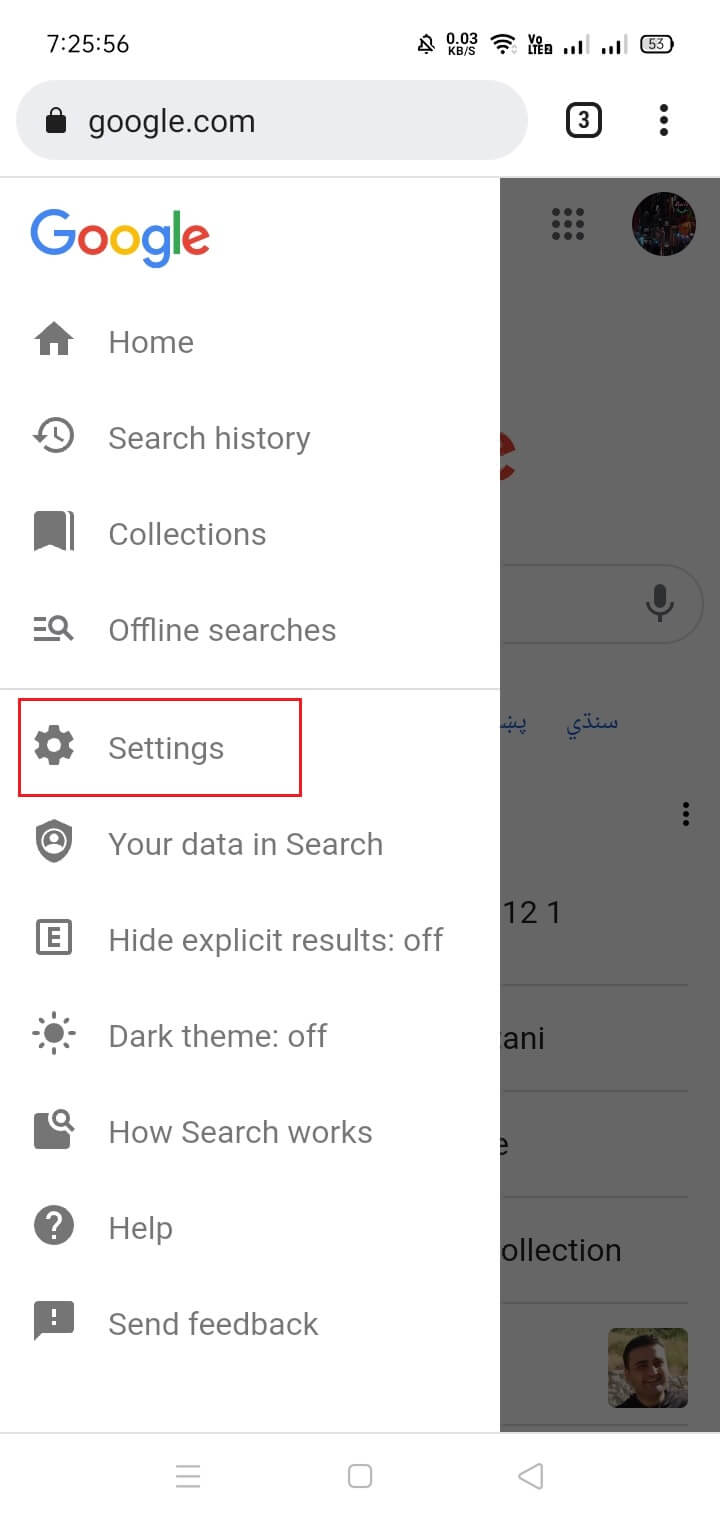The image is a screenshot taken from a mobile device displaying a Google.com page. At the top, the search bar prominently shows "Google.com," and below it, the distinctive Google logo is visible in its characteristic multicolored letters. Along the left side of the screenshot, there is a vertical list of icons, each associated with a specific function or category, with corresponding labels to their right.

Starting from the top, the first icon is a house, labeled "Home." Below it, a circular arrow icon indicates "Search history." Next, a ribbon symbol denotes "Collections," followed by a magnifying glass positioned over lines, representing "Offline searches." A faint gray line separates this section from the next.

The subsequent icon is a gear, labeled "Settings," which is notably highlighted by a hand-drawn red rectangle encircling it. Further down, a shield icon suggests "Your data in Search." The list continues downwards until it culminates with the "Send feedback" option.

On the far right of the screen, there is a gray shaded area that seems to be a pop-up box overlaying the lower part of the page. This detailed composition captures the user interface of a Google page on a mobile device, highlighting various navigational and functional elements available to the user.